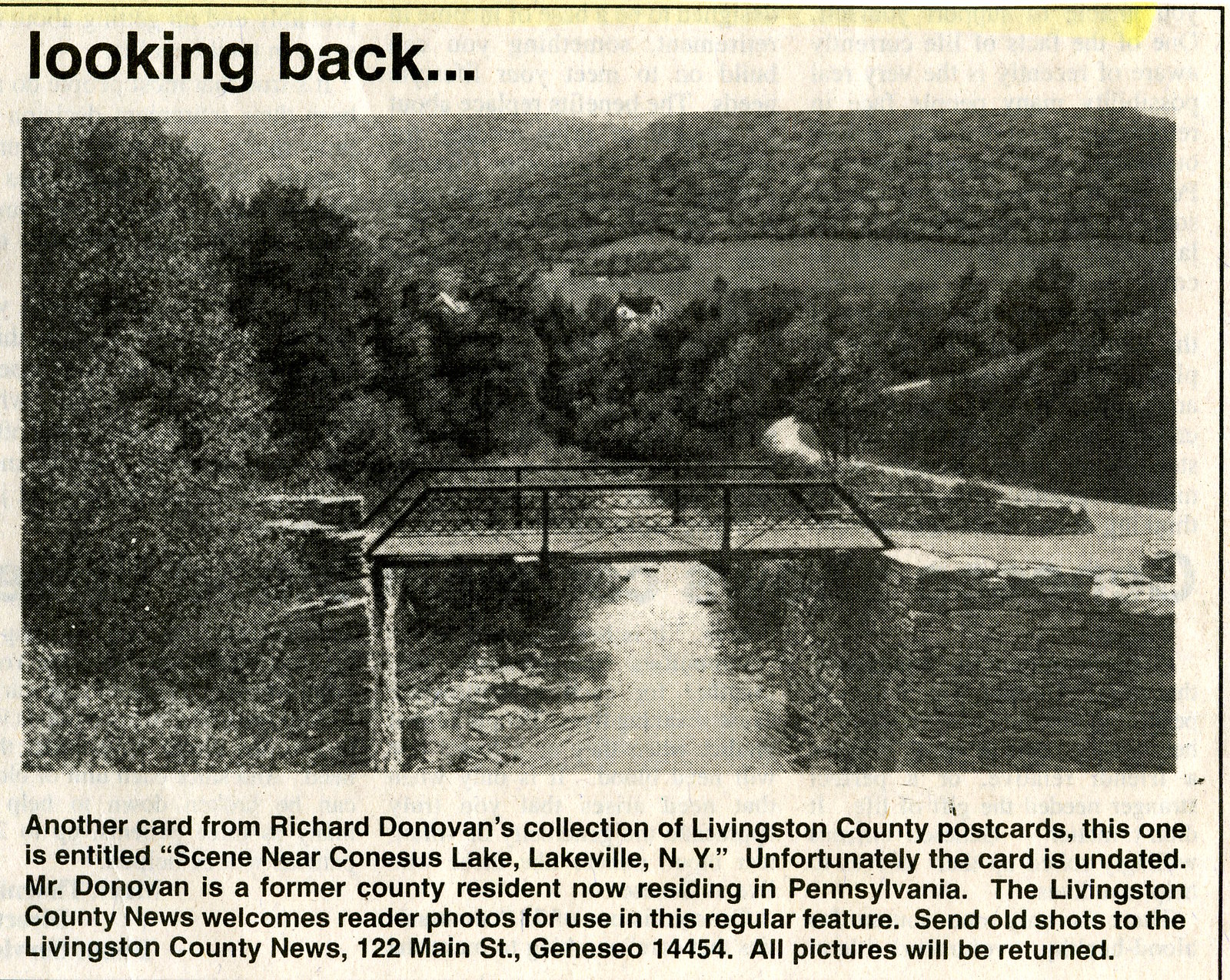Title: Looking Back

Description: This black-and-white image, framed by a black pinstripe border on its top and right sides, depicts a serene landscape. At the heart of the photograph is a sturdy bridge spanning a tranquil river, flanked by dense trees on both riverbanks. Beyond the trees, majestic hills or perhaps a mountain peak into the top right corner of the scene. Below the picture, a caption reads: "Another card from Richard Donovan's collection of Livingston County postcards. This one is entitled 'Seen Near Conesus Lake, Lakeville, New York.' Unfortunately, the card is undated." Accompanying this postcard snippet is a note indicating that Mr. Donovan, a former resident of Livingston County, now lives in Pennsylvania. The Livingston County News invites readers to submit their photos for this recurring feature, with assurances that all pictures will be returned.